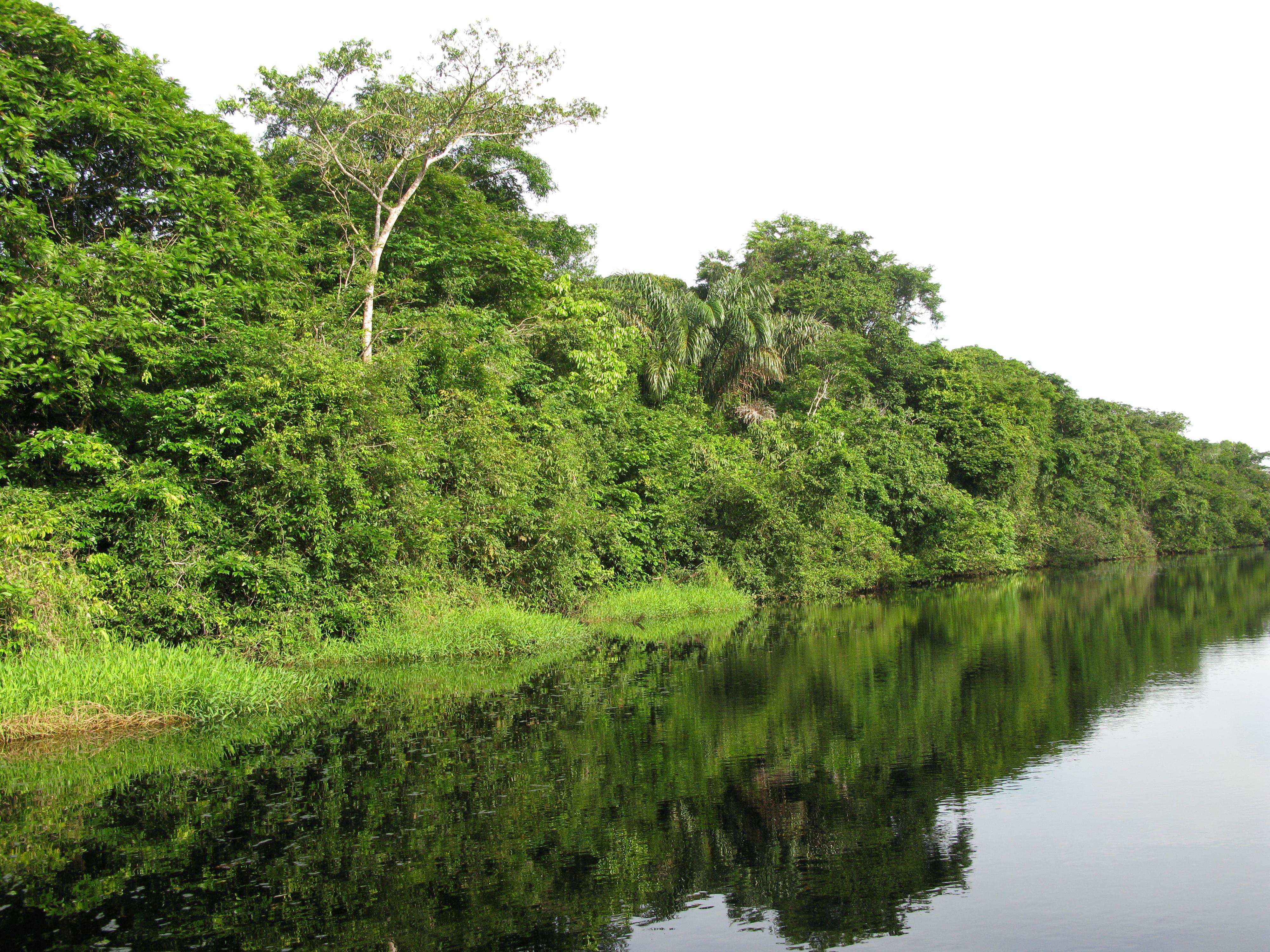The image captures an outdoor scene featuring a tranquil lake bordered by lush greenery. The lake’s surface is exceptionally still, creating a mirror-like reflection of the low shrubs, dense greenery, and trees that line the shoreline. From the upper left corner, tall trees and palm leaves extend skyward, tapering down to the lower right, where the water meets the edge of the photo. Among the foliage are visible shades of green interspersed with some brown patches of dead grass, and a distinct white-barked tree. The sky above the landscape is white and hazy, contributing to the serene and timeless quality of the scene, while it reflects as a light blue-gray hue in the lake below. The photo is rectangular, approximately six inches wide by four inches high, capturing this peaceful riverside or lakeside vista with no clear indication of the location or the photographer.